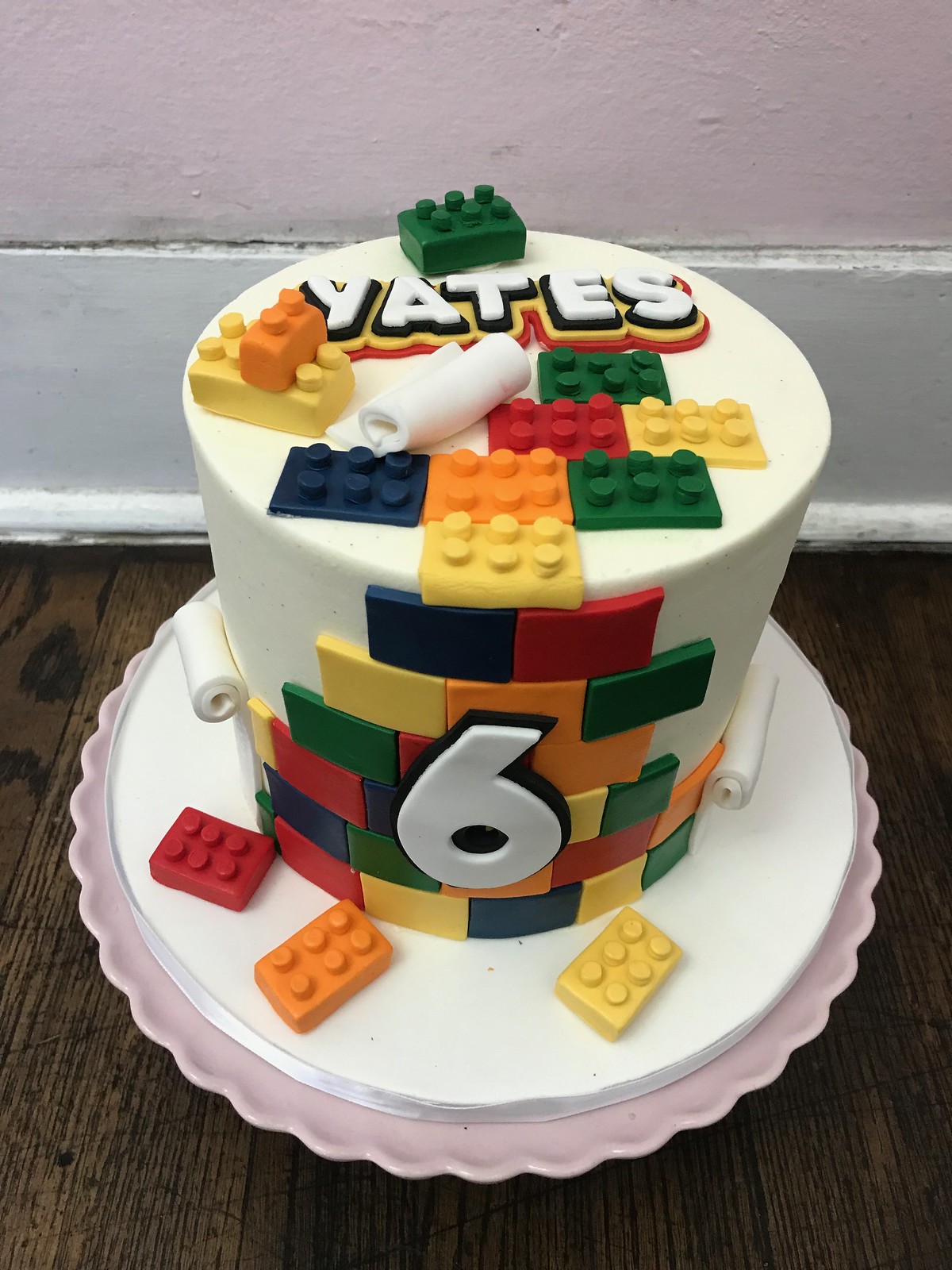The image depicts a tall, cylindrical birthday cake intricately designed with a Lego theme. The cake sits on a pink, scalloped cake platter, which rests on a dark wooden floor. The background consists of a white baseboard against a pink wall. The cake's exterior is covered in fondant and features a number "6" in white prominently displayed. Surrounding the number are various Lego-shaped decorations in green, red, yellow, orange, and dark blue, though these lack the characteristic Lego studs. However, atop the cake, similar Lego-like bricks with the distinctive studs are arranged, including a green brick, a yellow brick attached to an orange one, and a variety of other colors. At the very top, the name "Yates" is outlined in yellow and red, giving a 3D effect. Additionally, a piece of fondant is rolled up to resemble a scroll for added decor. The cake's detailed design gives the impression of a playful, birthday celebration theme centered around Lego bricks.